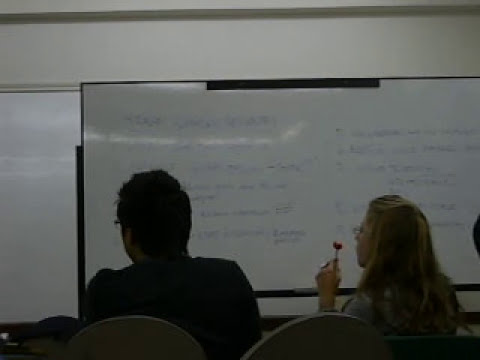In this detailed photograph of a classroom setting, two individuals are seated on gray folding chairs, facing a white dry erase board mounted on a white wall. The duo comprises a man and a woman, both wearing eyeglasses. The man, identifiable by his dark hair and dark jacket, sits with his back fully turned towards the camera, while the woman, who has blonde hair, is seen from a slight side profile. She is holding a lollipop in her hand. The dry erase board in front of them features text written in blue marker. This scene appears to be part of a presentation or lesson, with the focus on the subjects' attentive postures and the educational environment surrounding them.